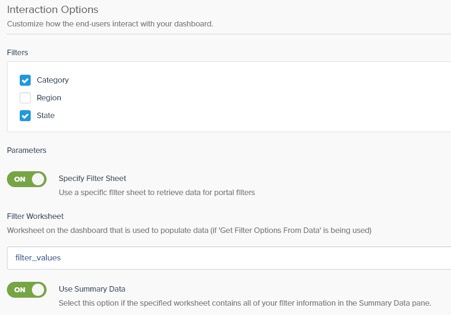**Detailed Caption:**

The screenshot displays the settings panel of an unspecified app, specifically focusing on interaction customization options for the user to adjust how end users interact with their dashboard. The panel is organized into several categories:

1. **Filters Section**: 
   - There are three filter options: "Category," "Region," and "State."
   - Both "Category" and "State" are enabled, indicated by a dark blue background with white check marks next to them.

2. **Parameters Section**:
   - An on-off toggle button labeled "Use Specific Filter Sheet to Retrieve Data for Portal Filters" is present and toggled on.

3. **Filter Worksheet Section**:
   - A description specifies that the filter worksheet on the dashboard is used to populate data, with the instruction:
     - `if ("get filter options from data")`.
   - Below this, there is an input box labeled with "filter_values."

4. **Summary Data Toggle**:
   - Another on-off toggle button is available, marked for "Use Summary Data." This option indicates that selected summary data will be used from the specified worksheet, and it is currently toggled on (green).

The overall interface has a light, clean design with a pale gray background and a lighter white shade for input fields. The fonts used throughout the panel are sans serif, enhancing readability. No additional details or app identifiers are visible in the screenshot.